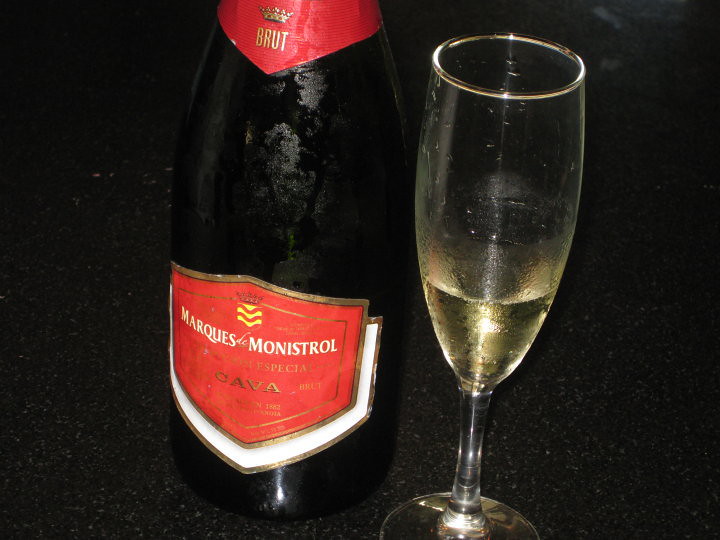The photograph showcases a close-up of a strikingly dark bottle, likely champagne or sparkling wine, positioned to the center left. The bottle is almost entirely black, obscuring any view of its contents, and adorned with two red labels bordered in gold. The top label features a gold crown above the word "Brut." Below, a broader cherry red label displays "Marquis de Monastrol" in white and "Cava" in bold gold at the bottom, with additional gold text partly obscured by lighting. The bottle sits on what appears to be a black granite countertop speckled with white.

To the right of the bottle, a champagne flute—filled about 20-30% with a golden-hued liquid—complements the scene. The flute is delicate, with a thin stem and droplets of condensation around its rim, adding a touch of elegance. The overall composition, set against the sleek, speckled black granite, exudes sophistication and a hint of mystery.